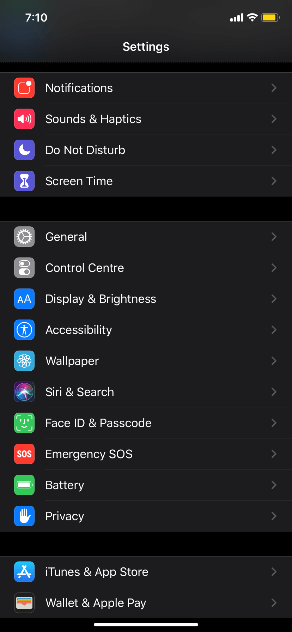The image captures the main settings screen of an iPhone, displayed in dark mode, with a black background. The top of the screen prominently displays "Settings," indicating the user is in the main settings menu. Below the title, various setting categories are listed in white text, each accompanied by distinct icons. These categories include: 

- **Notifications**
- **Sounds & Haptics**
- **Do Not Disturb**
- **Screen Time**
- **General** (highlighted with a gear icon)
- **Control Center**
- **App Store**
- **Wallet**
- **Emergency SOS** (indicated by an "SOS" icon)
- **Battery**
- **Privacy**

The iPhone's status bar at the top shows the time as 7:10, with a nearly full battery, full cellular bars, and a strong Wi-Fi connection. This interface is typical of iOS, whose design remains relatively consistent across different versions. The dark mode feature casts the entire background in black, enhancing the white text and icons' visibility. Icons further enhance the settings, such as an accessibility icon resembling a Vitruvian man and Siri’s signature swirling crystal ball-like symbol.